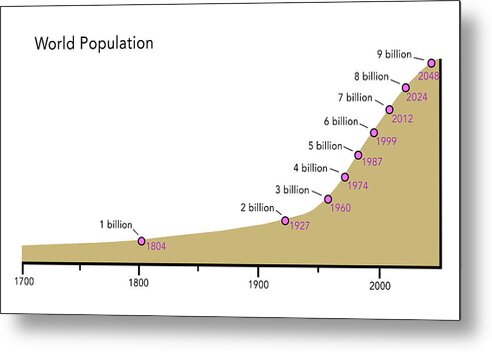The image is a detailed line chart against a white backdrop, titled "World Population" in the top left corner. The x-axis displays dates ranging from 1700 to beyond 2000, with significant markers at 1700, 1800, 1900, and 2000. Measuring increments are present, and key population figures are marked with pink dots. The line, which is beige or brown in color, indicates population growth, rising sharply especially from the mid-1900s onward. The chart highlights significant milestones: 1 billion in 1804, 2 billion in 1927, 3 billion in 1960, 4 billion in 1974, 5 billion in 1987, 6 billion in 1999, 7 billion in 2012, 8 billion in 2024, and an estimated 9 billion by 2048.